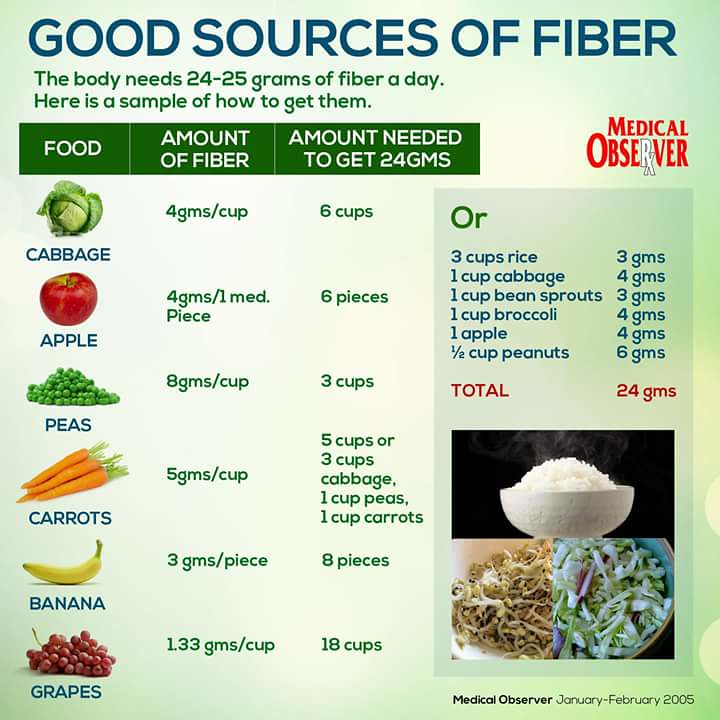The image depicts an informational chart titled "Good Sources of Fiber," which highlights the daily fiber requirement for the body—24 to 25 grams. The chart provides detailed examples of how to meet this requirement using various foods. For instance, cabbage provides 4 grams of fiber per cup, requiring 6 cups to meet the daily fiber needs, while an apple offers 4 grams, peas supply 8 grams per cup, carrots give 5 grams per cup, a banana has 3 grams per piece, and grapes have 1.33 grams per cup. Alternatively, the chart mentions that 3 cups of rice equals 3 grams of fiber, 1 cup of bean sprouts offers 3 grams, 1 cup of broccoli contains 4 grams, 1 apple gives 4 grams, and half a cup of peanuts contributes 6 grams. 

Visual representations include images of cabbage, apple, peas, carrots, banana, and grapes, each annotated with their corresponding fiber content and the quantity needed to achieve 24 grams. The visual elements are organized with the food items and their fiber amounts written in white on a green background. The chart also includes additional notes like "Medical Observer, January to February 2005" written in red and white, with the 'R' in "Observer" stylized as an RX, suggesting a health-related context. A light pale green background provides a cohesive backdrop, while a separate section features a steaming bowl of white rice, bean sprouts, and cabbage salad. This chart appears to be a page from a magazine named "Medical Observer."